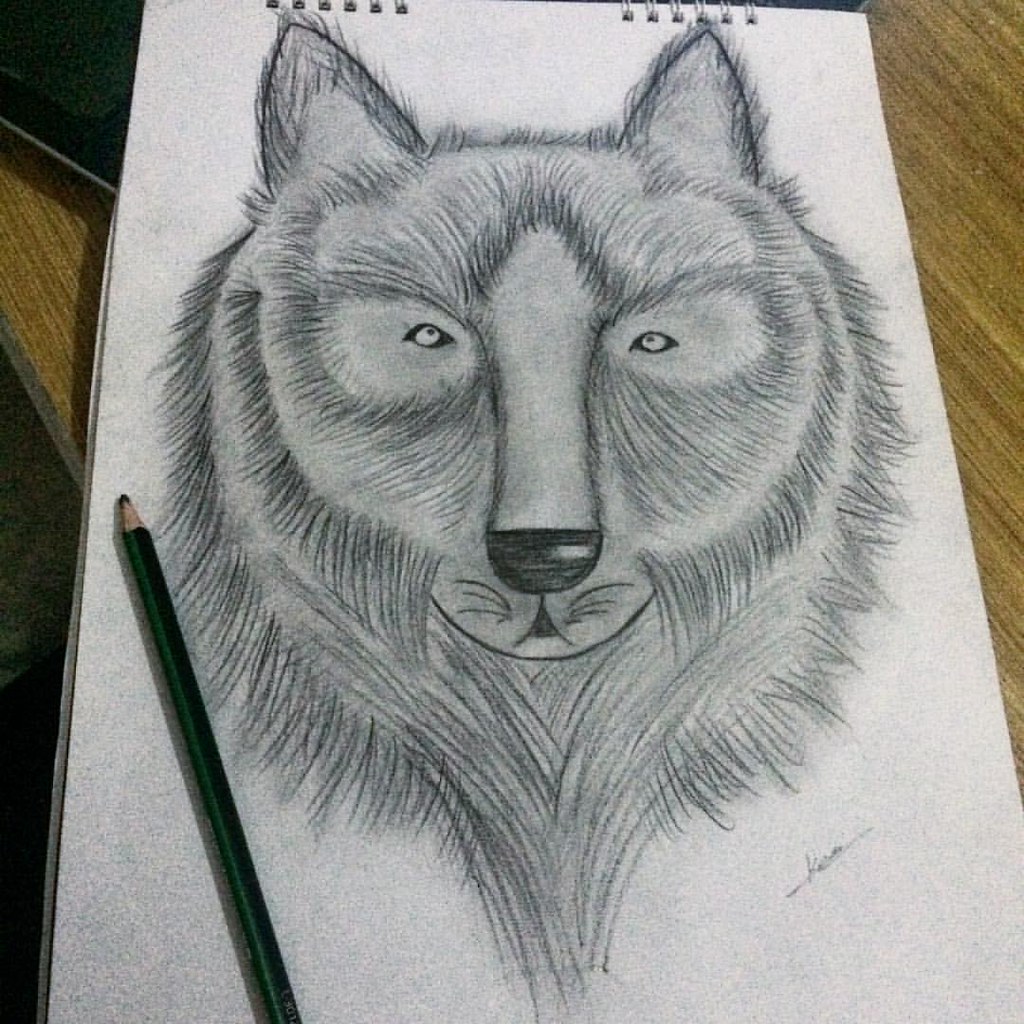This detailed charcoal pencil drawing showcases the head of an animal that is ambiguous in nature, resembling both a bear and a wolf. The head's cylindrical structure and v-shaped outline add to the complexity of its identification. Two pointed ears sit atop the head, also rendered in rich charcoal tones. The streaks of fur, meticulously detailed, cascade in various directions across the face and collar, enhancing the texture and depth of the piece.

The eyes are small and symmetrically positioned, giving the animal a focused yet enigmatic expression. The nose, distinctively oblong with a blackened tip, leans toward the characteristics of a bear. Set against the white paper, the piece captures both the softness of fur and the stark contrast of shadows. A signature, located in the lower right corner, is penned in visible black color pencil, marking the artist's completion of this evocative artwork.